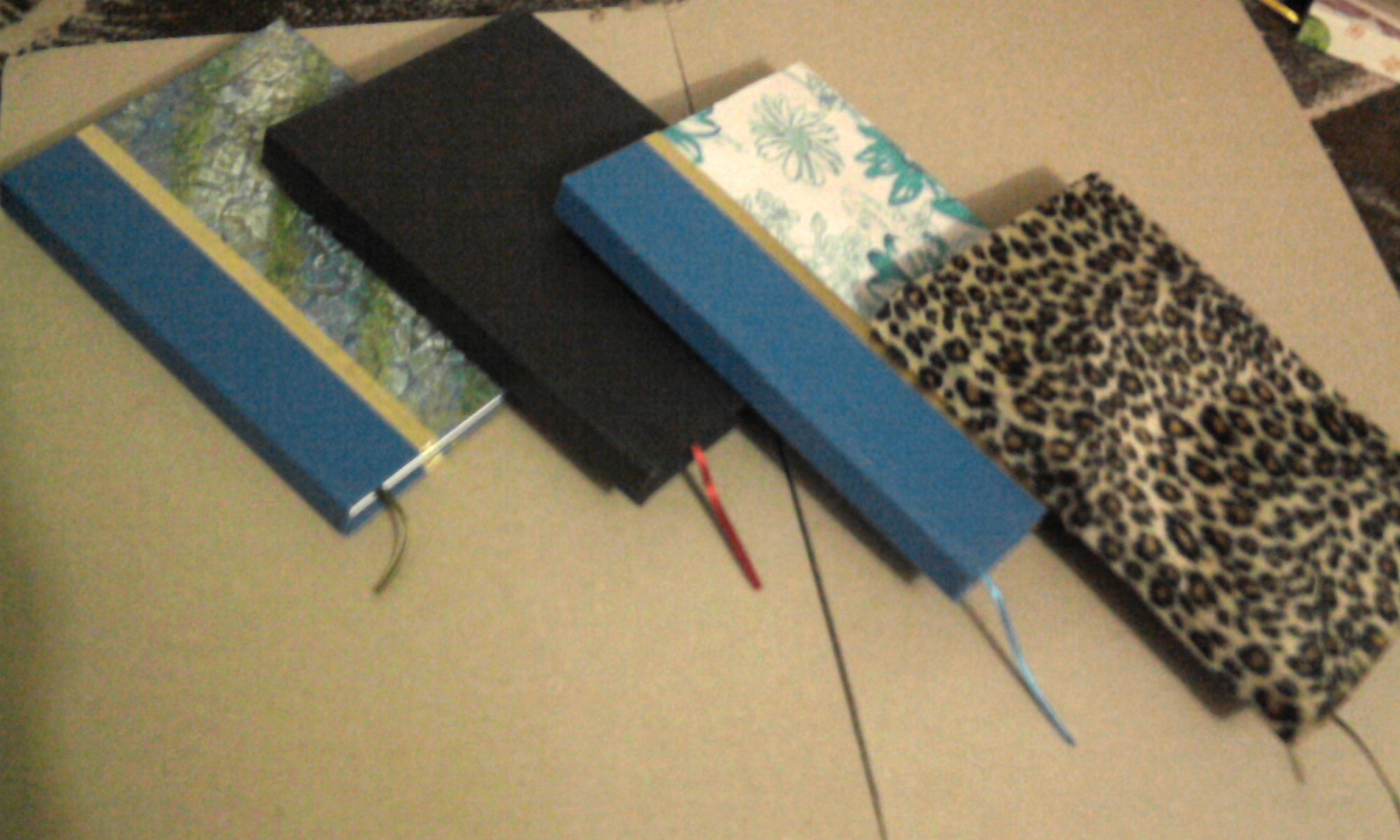This is a detailed color photograph taken indoors of four overlapping journals arranged from the upper left-hand corner to the lower right on a light brown, possibly beige, surface that doesn't occupy the entire frame. The bottommost journal features a leopard print cover. Above it, a journal with a dark blue spine and a light background adorned with blue and white flowers is placed. Next in the sequence is an all-black journal. The topmost one, on the far left, has a blue spine with a yellow stripe and a cover displaying a vibrant marbled design in shades of blue, green, and yellow. Each journal is equipped with a thin ribbon bookmark extending from the bottom near the spine. The background includes black areas on both the top left and top right corners of the image.